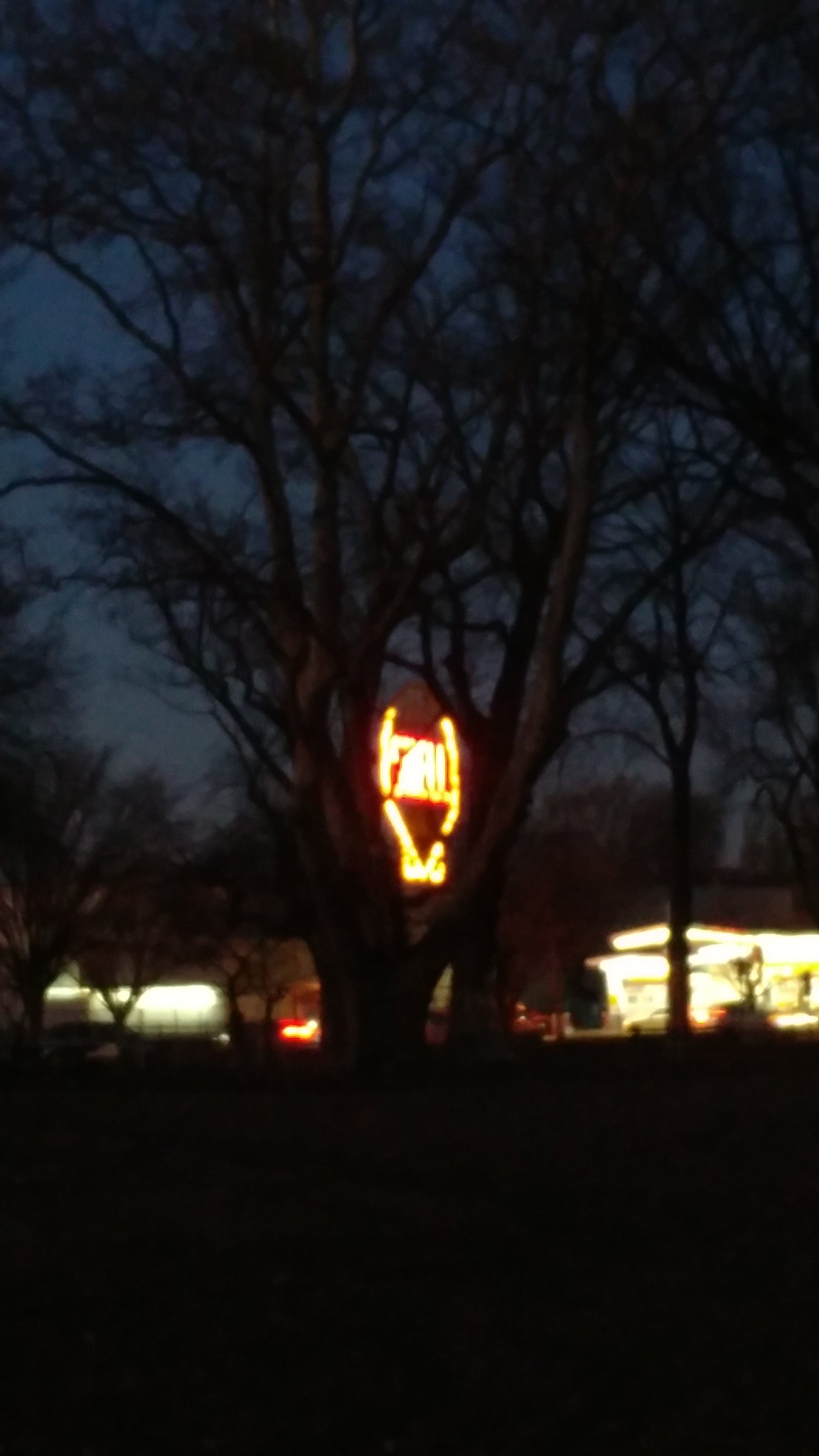This image captures a blurry nighttime scene through the branches of trees. In the foreground, a tree is partially visible. The background features a well-lit area that could either be houses or businesses, although the blur makes it difficult to discern. A neon sign, which might be an illuminated stop sign, stands out distinctly, casting a glow. The image also reveals several cars in the background, likely indicating an active area. The sky suggests it is just after sunset, with the majority of the lower portion of the picture shrouded in darkness. Despite the lack of clarity, the overall impression is that of a lively, albeit hazy, urban nightscape.